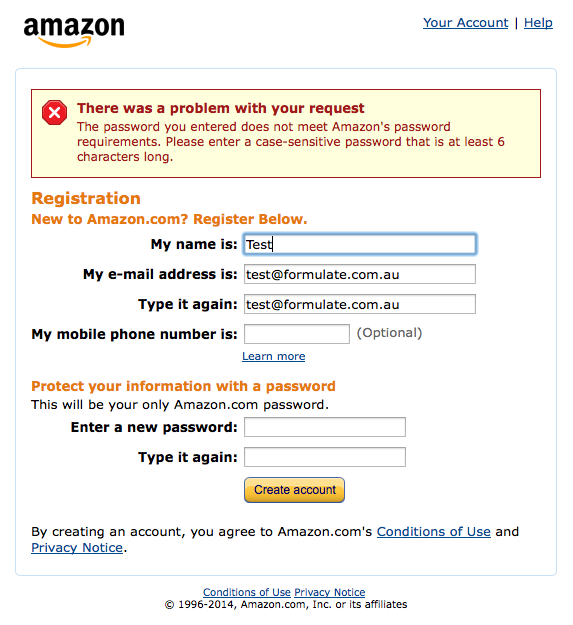This is a detailed screenshot from the Amazon.com registration page. At the top left corner, "Amazon" is prominently displayed. On the top right, the options "Your Account" and "Help" are visible. 

A yellow rectangle with a red border alerts the user with the message, "There was a problem with your request. The password you entered does not meet Amazon's password requirements. Please enter a case-sensitive password that is at least six characters long."

Below this, the user is prompted to fill in registration details under "New to Amazon.com? Register below." The fields are populated with placeholder information: "My name is," followed by "test." The email address field is filled with "test@formulate.com.au," repeated again in the confirmation email field.

The mobile phone number section is blank, with "optional" and "learn more" adjacent to it.

Next, users are instructed to "Protect your information with a password." Below this prompt, two blank boxes are provided for entering and confirming a new password.

At the bottom of the form, a large orange rectangle with the text "Create account" in black writing stands out. A disclaimer at the bottom reads, "By creating an account, you agree to Amazon.com's Conditions of Use and Privacy Notice." Links to "Conditions of Use" and "Privacy Notice" are provided. The footer also includes a copyright notice: "© 1996-2014, Amazon.com, Inc. or its affiliates."

The screenshot does not contain images of people or animals, focusing solely on the registration form.